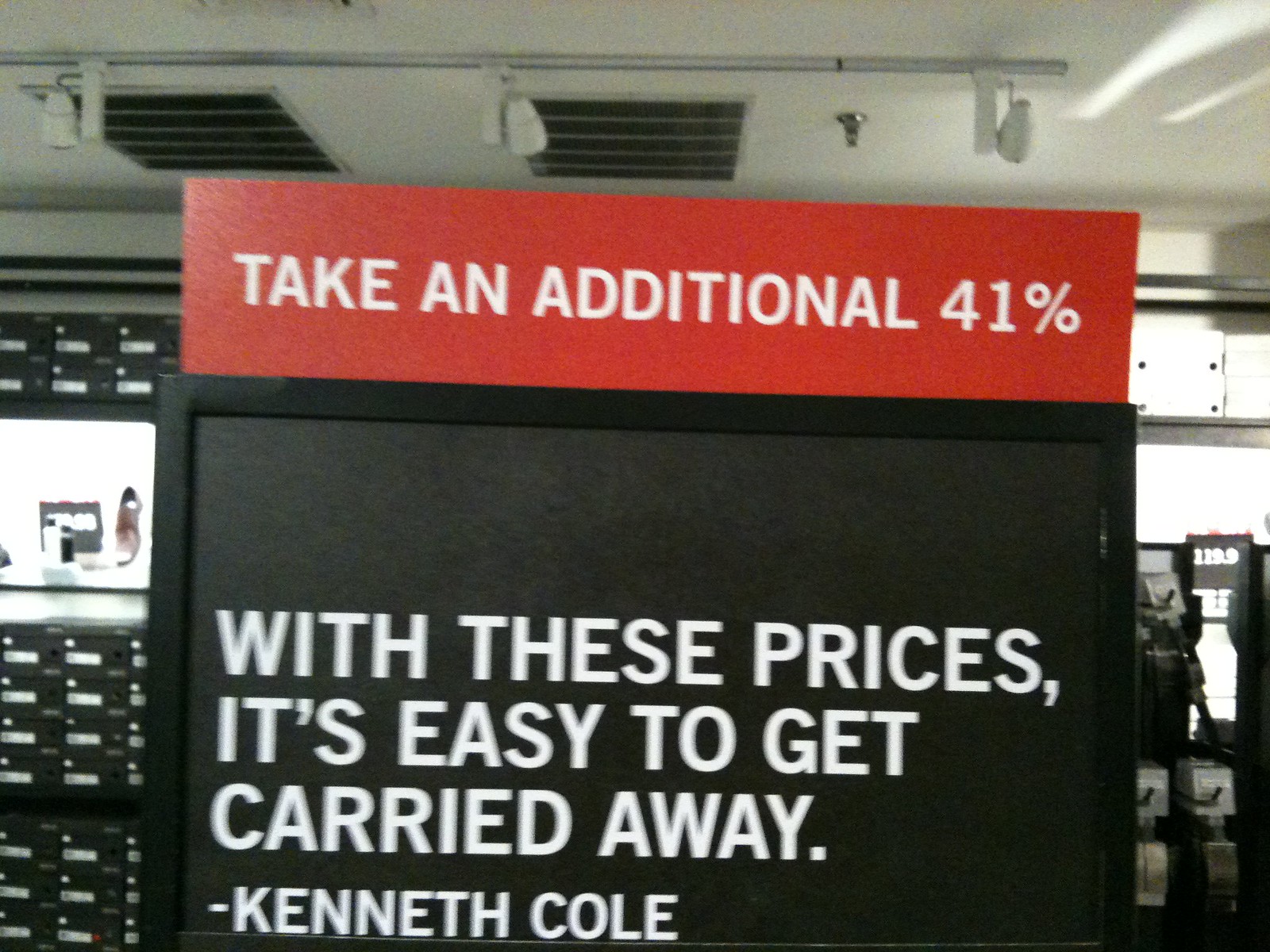The photograph captures a promotional sign prominently displayed within what appears to be a store, likely a shoe store or shoe department. The sign, viewed from the front, is large and square, featuring a black background with white text. At the top, a red rectangular section announces in white lettering, "Take an additional 41% off." Below this, the main section of the sign reads, "With these prices, it's easy to get carried away," attributed to Kenneth Cole. The environment includes a white ceiling equipped with six spotlights and two commercial air conditioning intake vents. Display racks can be seen below the sign, with boxes of shoes on the left and other display racks, potentially for socks, on the right, reinforcing the retail setting.